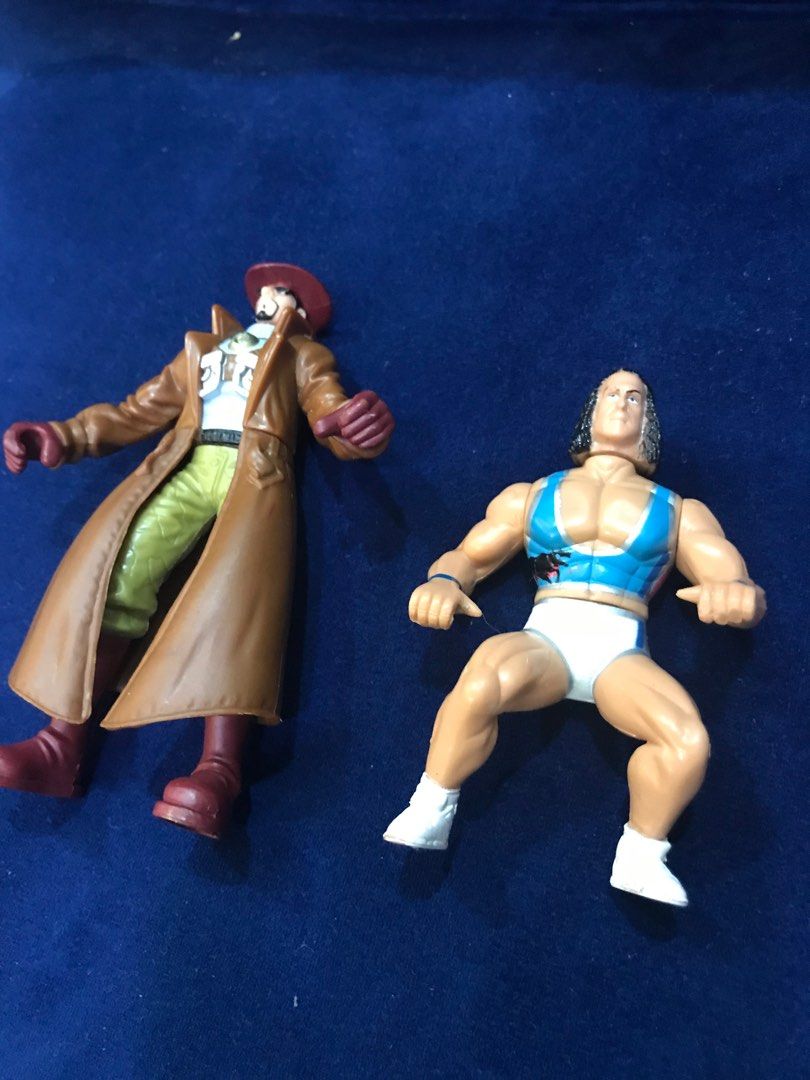In this color photograph, two action figures are lying on a blue surface, which could be either a tablecloth or a carpet. The first figure, located on the left, is dressed in a long brown trench coat, a brown Indiana Jones-style hat, green pants, a black belt, and brown boots. He also has brown gloves with grasping hands positioned outward at a 45-degree angle from his body. This figure appears to be looking towards the upper left corner and boasts a distinctive black beard or goatee. Underneath his trench coat, he wears a white shirt with a protective shield on the chest. 

The figure on the right side embodies a wrestler with a highly muscular build, showcased by a tight blue tank top that reveals his bulging chest muscles. This figure is posed as if squatting, with bent knees and arms at his sides, palms downward, and thumbs pointed inward. He has long curly hair reminiscent of Bret Michaels, and his outfit includes very short white shorts and white high-top shoes. Together, these figures create a dynamic and visually detailed scene, highlighting their distinct yet complementary characteristics.